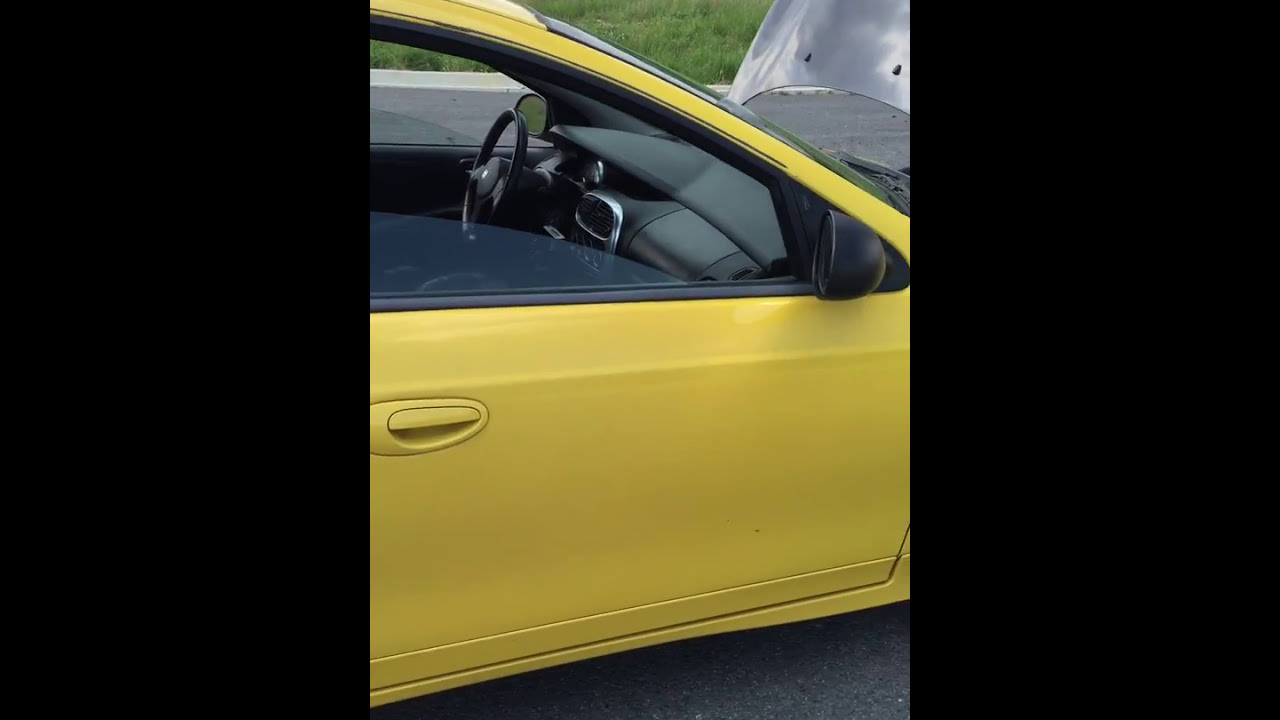The image is a full-color outdoor photograph bordered on the left and right by black panels, with no border on top. The central panel showcases a bright yellow car parked on a dark gray concrete surface. The car's passenger side window is rolled down about three-quarters of the way, revealing a black leather interior with a black steering wheel and front dashboard. The door handles are yellow, matching the car's exterior. The car's hood is open, exposing a dark gray metal piece jutting into view on the right side of the image. The side view mirrors are black, contrasting with the yellow body of the car. There is no passenger or driver inside the vehicle. In the background, green grass can be seen, suggesting the car is parked near a grassy area, possibly beside a road. The scene is still, with no visible text or action taking place.